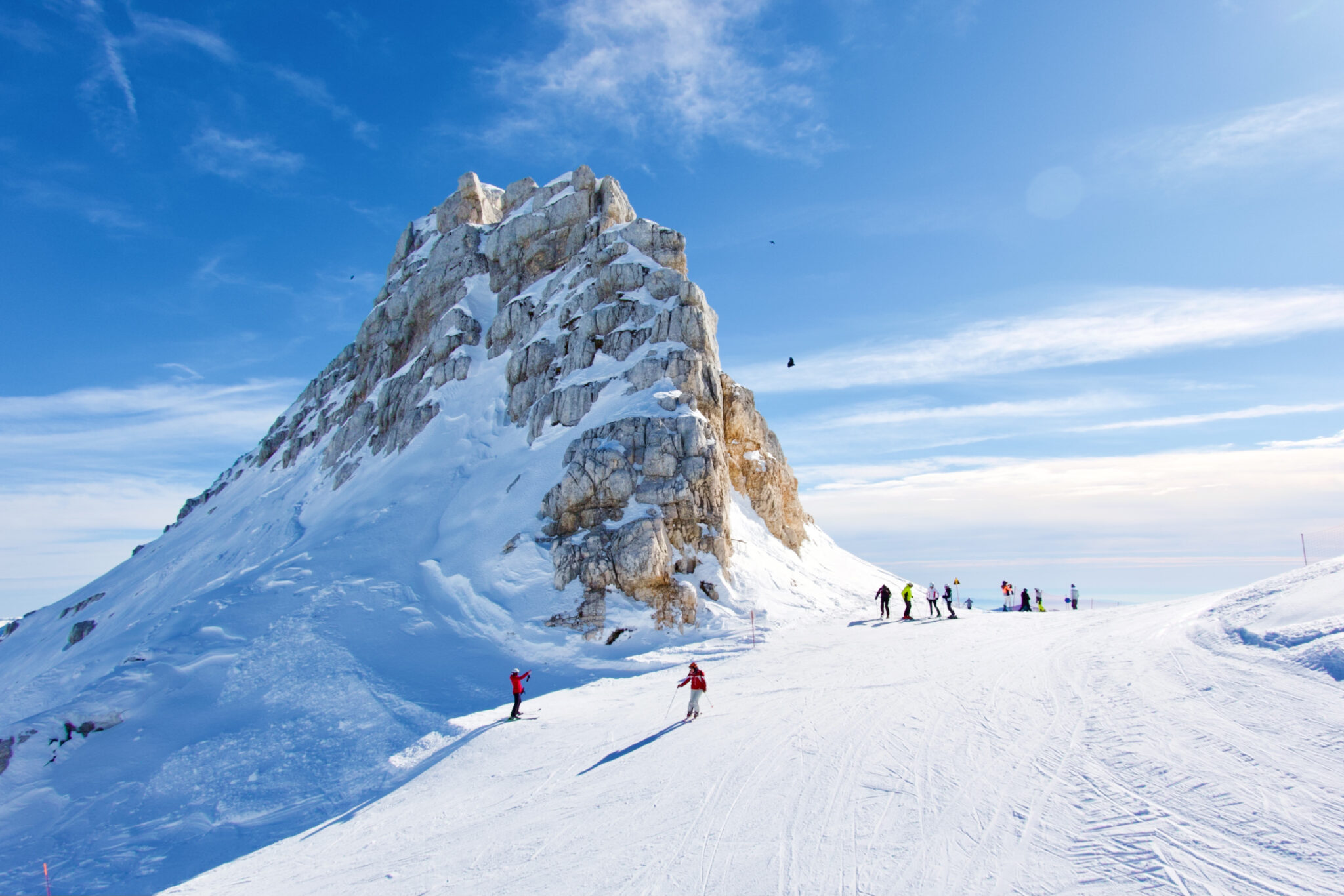This outdoor photograph captures a clear, sunny day on a picturesque ski slope. The bright blue sky, dotted with light, wispy clouds, serves as a stunning backdrop. In the foreground, a skier in a red jacket and white pants begins to descend the snow-covered slope. To the left, a rugged mountain peak emerges prominently against the sky, its summit lightly dusted with snow while its base is buried in a thicker layer. Nearby, another individual in a red jacket appears to be taking a photograph of the skier. Further up the slope, two groups of skiers can be seen: one preparing for their descent, and another already skiing down in the opposite direction. In the distance on the right, numerous figures dot the landscape, adding a sense of scale and activity to the winter scene.